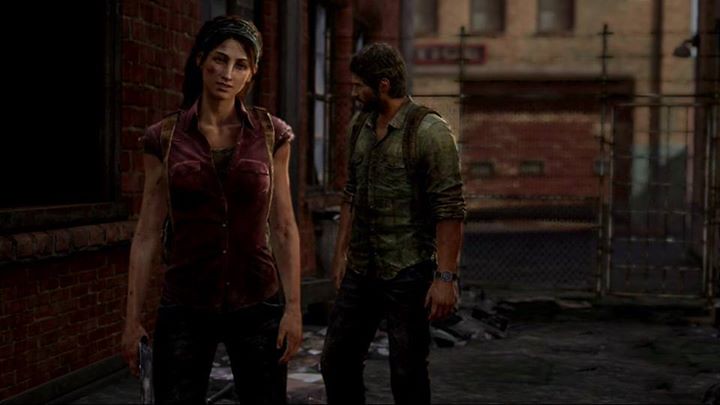This is a screenshot from a video game capturing an intense moment in a gritty, urban alleyway. Positioned in the foreground on the left side is a woman, her appearance smeared with dirt, signifying the harsh environment. She is equipped with a leather-strapped backpack that secures around her shoulders and under her arms. The woman is dressed in a red, short-sleeved shirt featuring two front pockets, paired with black pants. In her hands, she firmly grips a gun, indicating they are likely in a dangerous situation.

Behind her, to her right, stands a man equally smudged with grime, also wearing a similar strapped backpack. The background reveals an old brick building, adding to the dilapidated atmosphere. A metal chicken wire fence and a metallic door lie directly behind them, while across the alley, an aged garage door is visible. Scattered around are pieces of trash, further contributing to the scene's overall sense of decay and abandonment.